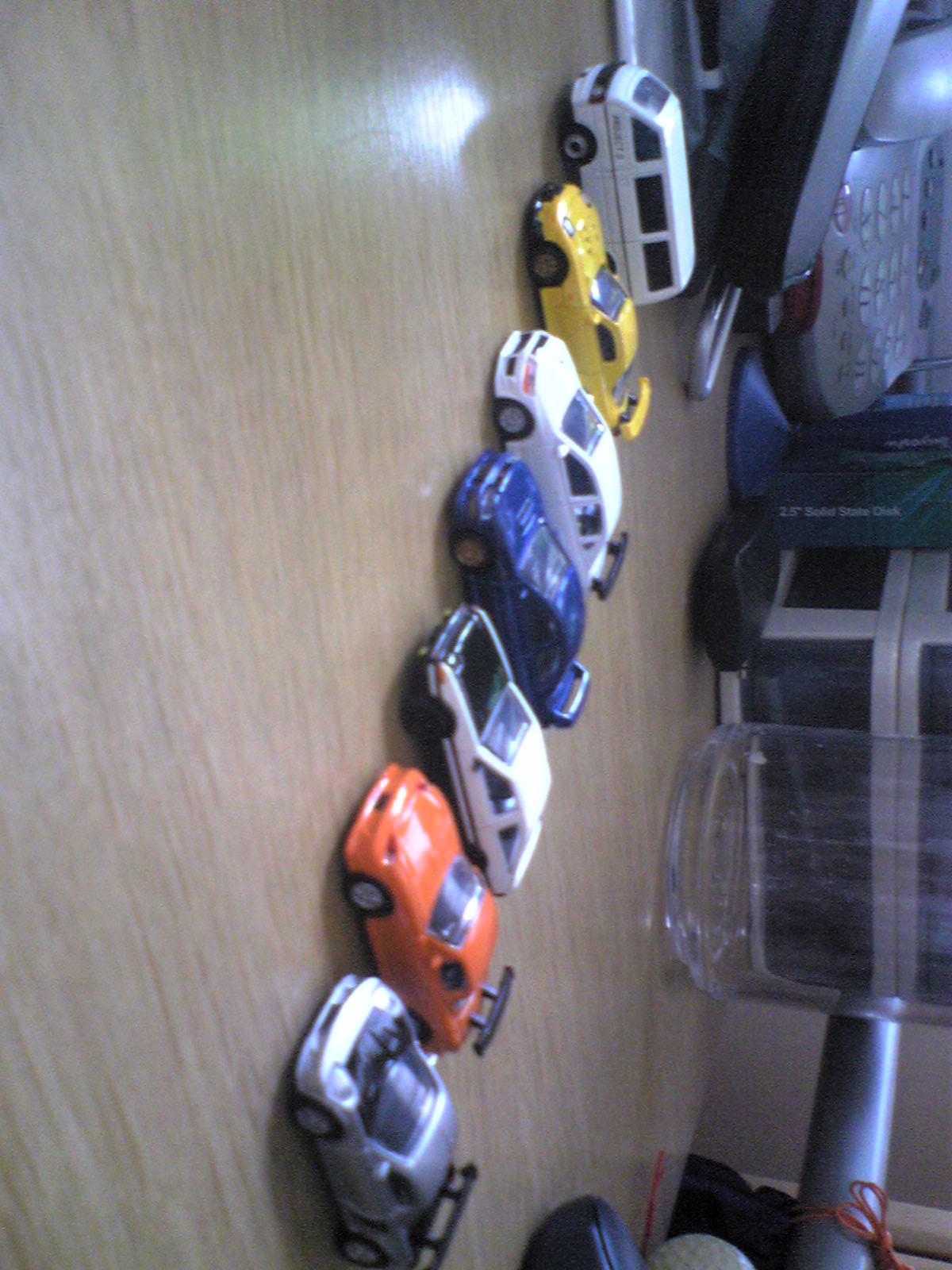This is a vertically rotated close-up photograph of seven small toy cars, positioned on a wooden surface with noticeable wood grain. The collection includes six sports cars and one Volkswagen-style van. Among the cars, five feature spoilers. The cars, aligned in a row, showcase a variety of colors: silver, orange, white, cobalt blue, school bus yellow, and a distinctive white van with smoky windows and a musclehead-style white car with a black hood. The background reveals additional desk items, including a telephone with an answering machine, plastic container drawers, a clear glass beaker, a computer monitor, and a mouse. Some white, indiscernible lettering, possibly on a keypad, can also be seen. Reflections from the light can be observed on the cars and the wooden surface.